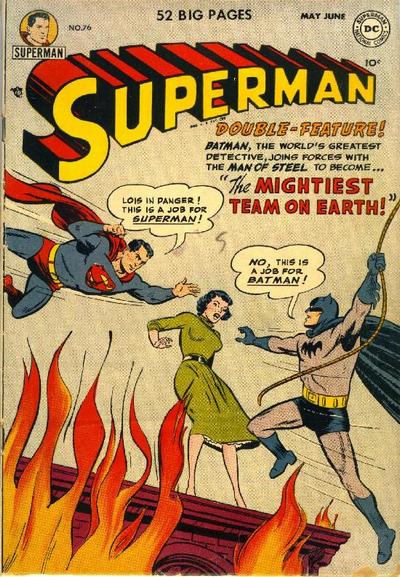This vintage comic book cover features Superman prominently, capturing the essence of classic superhero action. In the upper left corner within a yellow circle, we see Superman’s face with his iconic black hair and a glimpse of his red super suit. Just below, in a white rectangle, the text reads “Superman,” followed by the issue number "76." Central to the cover, large black letters announce "52 Big Pages,” flanked on the right by “May-June” and the DC Comics logo, with “10 cents” below. The word “Superman” is boldly displayed in imposing yellow text with a red shadow, adding a three-dimensional effect.

In a dynamic scene, Superman, in his blue suit with red tights and cape, featuring the famous red 'S' on a yellow shield, is depicted flying to the rescue. His thought bubble reads, "Lois in danger! This is a job for Superman!" Below him, Batman, wearing his gray and black bat suit, complete with a mask and golden utility belt, holds a rope in his right hand and exclaims, "No, this is a job for Batman!" Both heroes are converging to save Lois Lane, who stands terrified on the edge of a red building engulfed in red and yellow flames. Lois is dressed in an olive green dress, adding to the dramatic tension of the scene.

Below Superman, the text in orange states "Double Feature!" followed by “Batman, the world’s greatest detective joins forces with the Man of Steel to become,” with the phrase “the MIGHTIEST TEAM ON EARTH!” in bold red letters. The entire cover is set against a background with gray and white patterning, enhancing the vintage feel of this action-packed comic book.